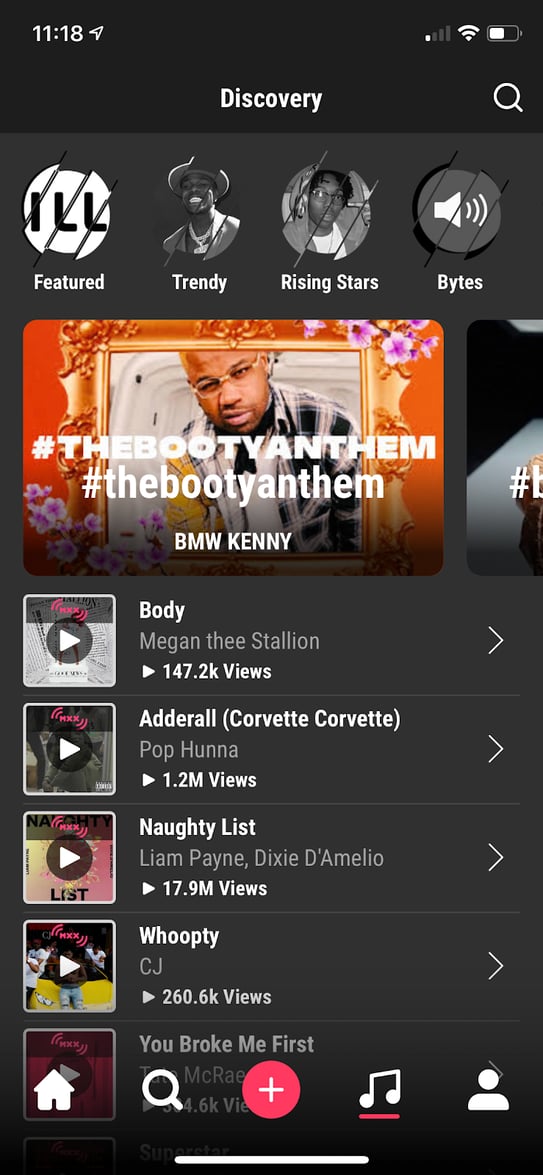The top section of the image shows various status indicators: it reads "11:18" with one out of four bars for signal strength, a Wi-Fi icon, and a 50% battery marker. Below these indicators, the screen displays the word "Discovery" along with a search magnifying glass icon. Under this, there are several category titles including "IOL Feature," "Trendy," "Rising Stars," and "Bytes."

The main content showcases popular music tracks. The first track is "The Booty Anthem" with the hashtag #TheBootyAnthem, attributed to BMW Kenny. Below this, additional tracks include "Body" by Megan Thee Stallion with 147.2k views, "Adderall (Corvette Corvette)" by Pop Hunna with 1.2 million views, "Naughty List" by Liam Payne and Dixie D'Amelio with 17.9 million views, and "Whoopty" by CJ with 260.6k views.

Another track titled "You Broke Me First" is partially visible, but the name is obscured by a red circle with a plus sign in the middle and a search icon.